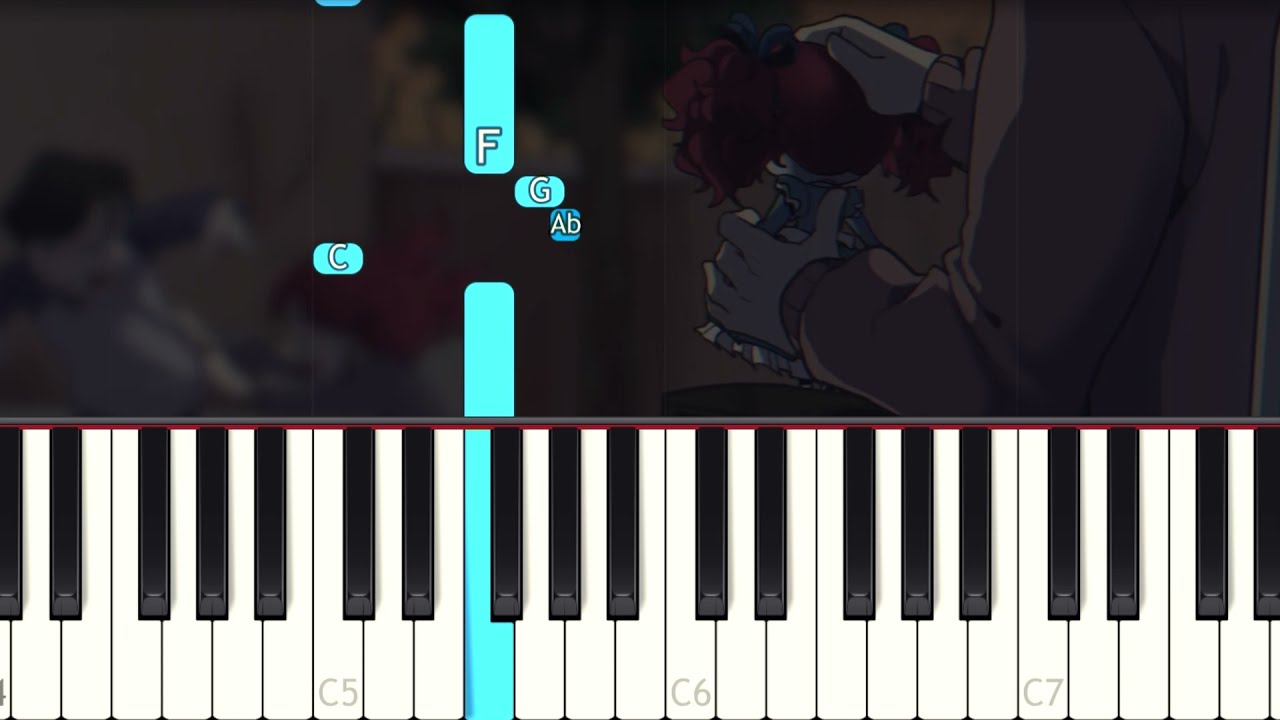The image is a detailed, color illustration in a landscape orientation, featuring a top-down view of a piano keyboard occupying the bottom half of the image. Several keys are labeled with their octaves, notably C5, C6, and C7. The top half of the image resembles a video game interface akin to Guitar Hero, with color-coded notes labeled with letters such as C, F, G, A, and B in turquoise and blue, falling in lines towards their corresponding piano keys. In the top-right corner, part of a character from the chest to the waist is visible, wearing a jacket and holding a doll with red pigtails and a blue outfit. The overall style is an illustrative combination of educational software and gaming elements.